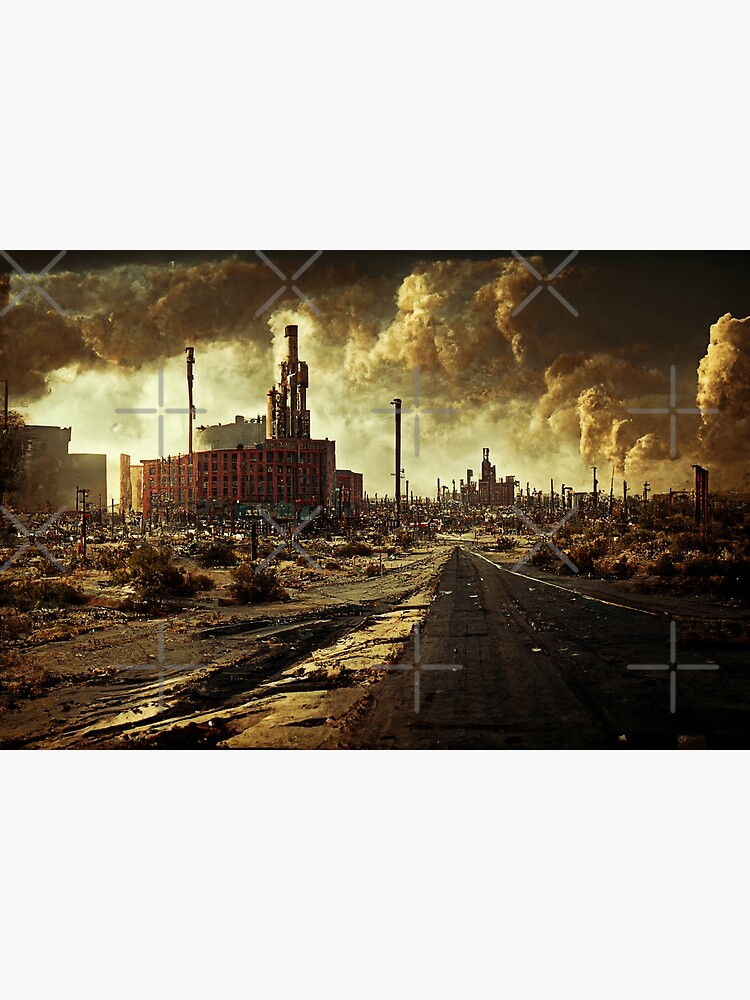The horizontal and rectangular, full-color digital artwork depicts a post-apocalyptic scene dominated by severe pollution. The entire top portion of the image is filled with billowing clouds of white, brown, and black smoke emitted from numerous factory smokestacks, giving the sky a heavily smoggy appearance with an amber-yellow tint, almost resembling a war zone. In the lower right corner, an old, blacktop road stretches off into the distance, leading towards a city filled with tall, pipe-laden industrial buildings. This road is littered with debris and flakes, bordered by a barren landscape of dirt and desert-like sand, sporadically dotted with scrub brush and bushes in various greenish and tan hues. The lower left section of the image is similarly arid, featuring more barren dirt and scrub vegetation. To deter unauthorized use, the artist has overlaid the scene with light gray X's and plus signs as a watermark.